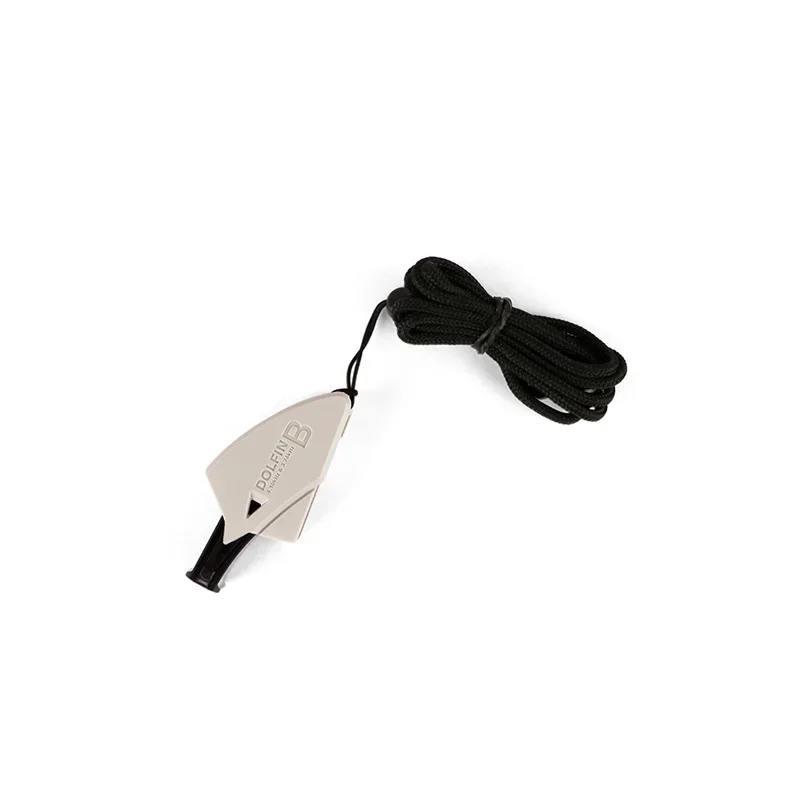The image depicts a small object with a sharp, triangular shape, likely made of a light gray or white plastic material. The background is entirely white, which highlights the object clearly. This object has a distinctive design, with one end resembling the tip of a balloon, black in color, where it seems one would blow into it. Along the body of the object, the word "DOLFIN" is inscribed with a prominent "B." A black cord is attached, wrapped neatly around the object and secured by a rubber band. The cord extends outward from a part of the object shaped somewhat like a sharp tooth or a V-shape sheath. This intricate setup suggests it might be an emergency blade or a multipurpose tool, where the cord and the sheath are essential components. The overall design and details, including the branding and structural elements, are the focal points of the image, with no other items present in the background.